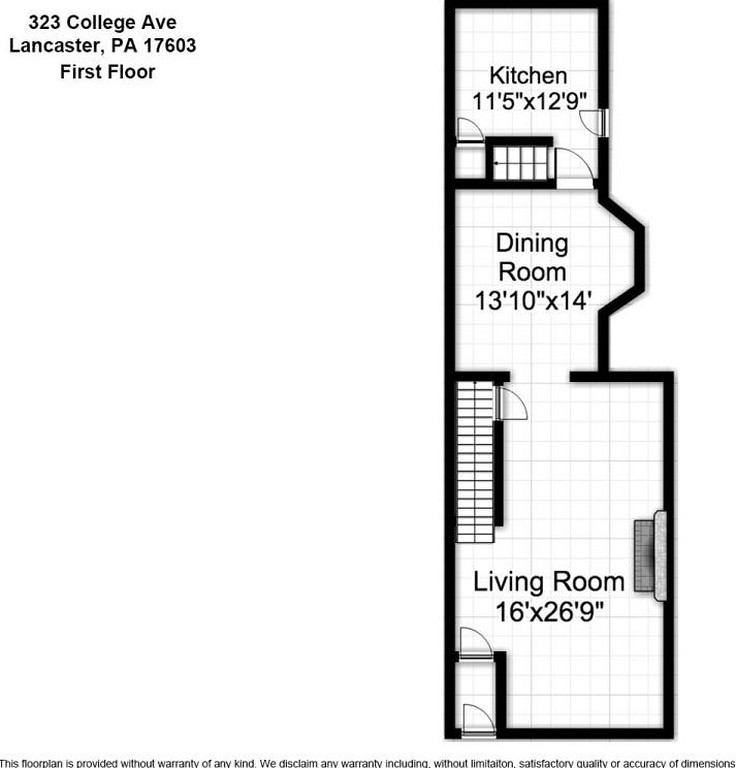This photo showcases a versatile, open-concept space that seamlessly integrates a living room, dining room, and kitchen. Located at 323 College Avenue, Lancaster, Pennsylvania 17603, this first-floor layout highlights a spacious living room measuring 16 feet by 26 feet 9 inches, making it the largest area. Adjacent to it is the dining room, which measures 13 feet 10 inches by 14 feet, while the kitchen spans 11 feet 5 inches by 12 feet 9 inches. The cohesive design of this multi-functional space offers both style and practicality, ideal for entertaining and day-to-day living.